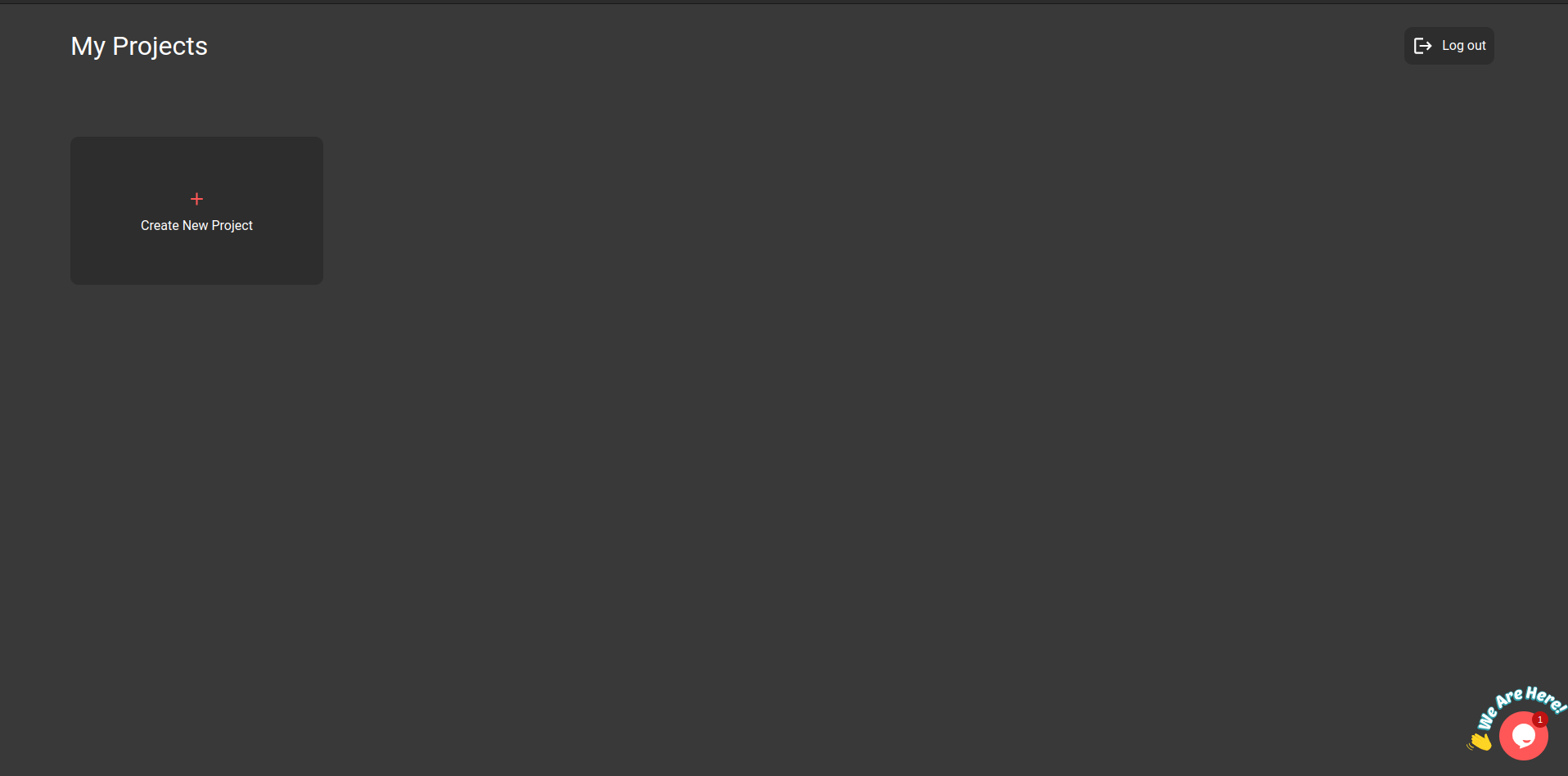This is a digital image showcasing a user interface with a solid medium gray background. Prominently featured is a perfectly rectangular shape. In the top left corner, the text "My Projects" is displayed. Opposite it, in the top right corner, is a small white arrow button indicating "Log Out." Below "My Projects," there is a tab titled "Create New Project," illustrated by a small black rectangle with a red plus sign. The text "Create New Project" is inscribed in white font above this icon. In the lower right corner, the phrase "We Are Here!" is displayed, hinting at a section or indicator within the interface.